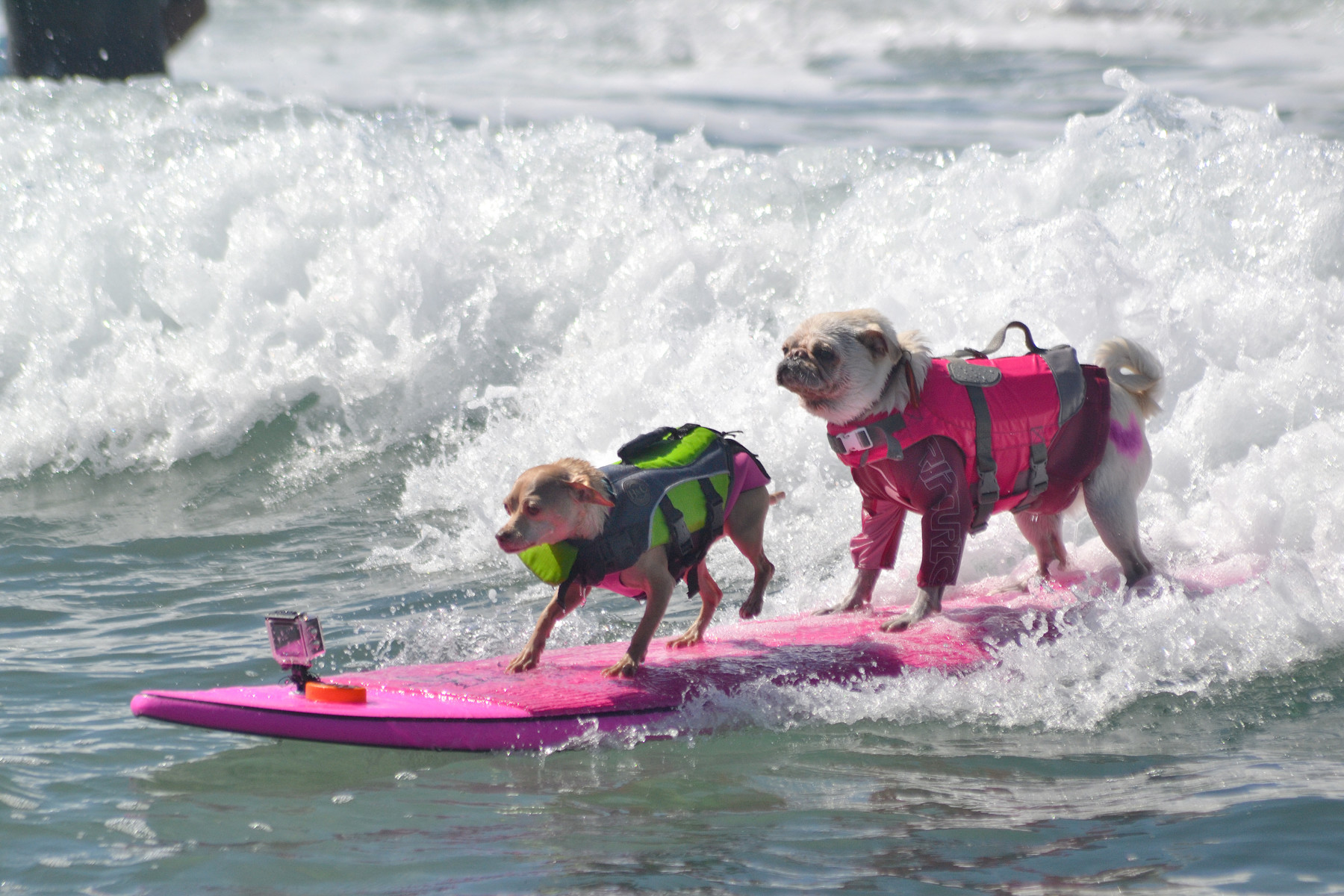In this entertaining and detailed photograph, you see two dogs skillfully riding a wave on a bright pink surfboard in the ocean. Both dogs are equipped with life jackets for safety. The smaller dog at the front is a skinny brown canine wearing a gray and neon yellow life jacket. Notably, its left hind leg is lifted, perhaps due to a mix of excitement and apprehension. Positioned behind is a larger, white pug, its curly tail peeking out from a pink and gray life jacket. 

The pug appears more stable, with all four feet firmly planted on the surfboard. A GoPro camera is mounted at the front of the surfboard, likely capturing this thrilling adventure. The scene is set against a backdrop of foamy waves breaking, suggesting the dogs are navigating through a substantial wave while heading toward the shore. To the top left of the frame, part of a person in a black wetsuit is slightly visible, possibly overseeing the dogs' surfing escapade. This outdoor shot perfectly captures the unexpected and charming moment of two dogs surfing, backed by the majesty of the ocean waves.